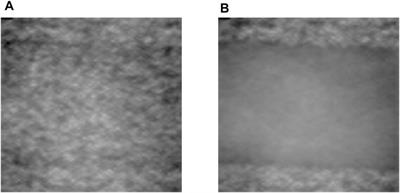The image features two perfectly square images set against an indistinguishable white background and labeled in the upper left corners: A on the left and B on the right. Both squares are gray, black, and white speckled textures, similar to an off-channel television static or a closely zoomed-in view of a rough surface like a stucco wall or cement. Image A manifests a consistently speckled and rough texture throughout. In contrast, Image B shares this speckled texture only in the top and bottom 20%, with a smoother, medium-gray area occupying the center. The visual disparity suggests a comparison of textural differences between the two images.